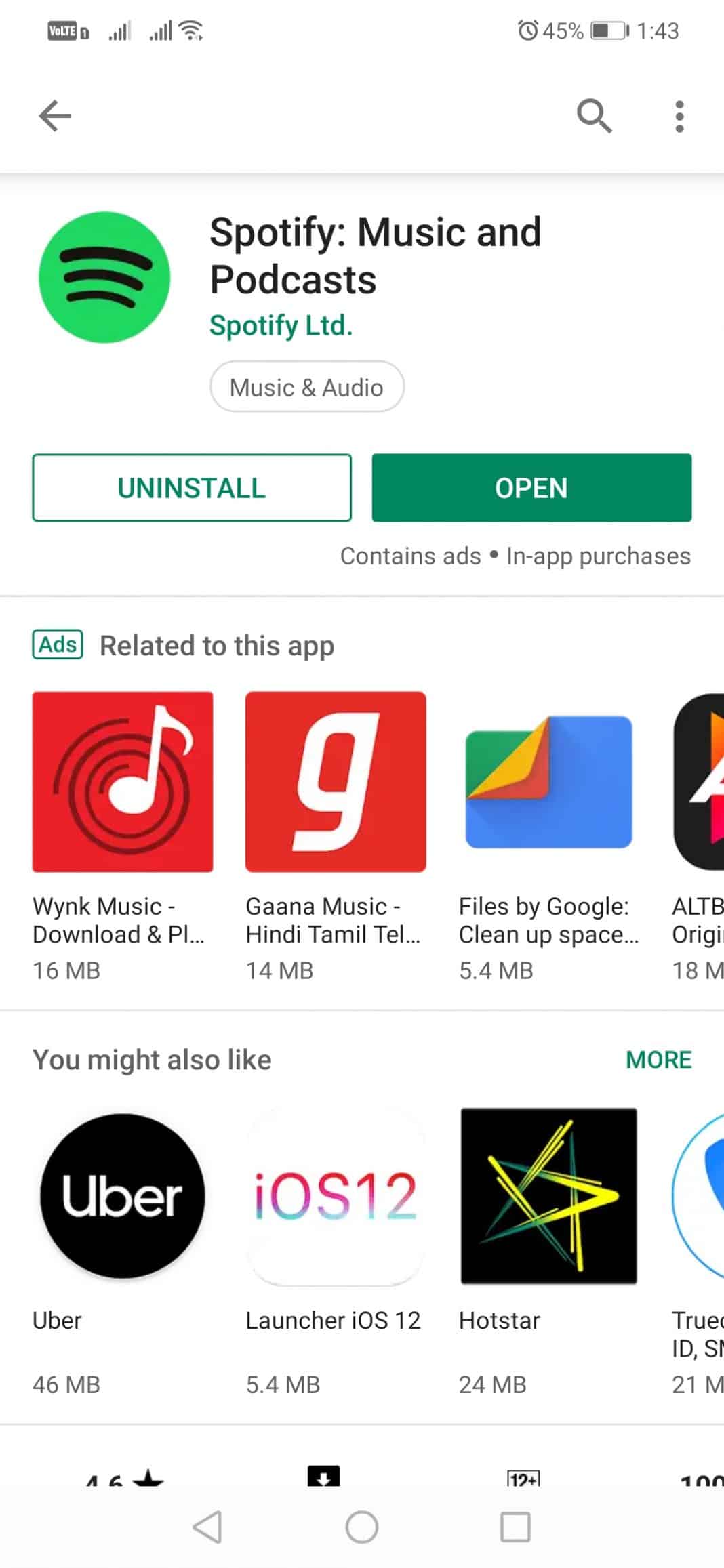The screenshot displays a smartphone with a 45% battery level. The screen shows the Google Play Store page for the "Spotify: Music and Podcasts" app developed by Spotify Ltd. The app's icon features the familiar green circle with three curved black lines. Below the app's name, there are buttons labeled "Music & Audio" and options to "Uninstall" or "Open" the app. 

Beneath these options, there's a section titled "Ads related to this app" which lists other music-related apps such as "Wynk Music" (16 MB, identified by a series of circles with a musical eighth note), "Gaana Music" (with a small lowercase "g" on a red background), and "Files by Google" (featuring the traditional multicolored icon).

The "You might also like" section suggests additional apps including "Uber" (with its black-and-white logo), "Launcher for OS 12," and an icon depicting a gold star on a black background, among others. Some app icons are partially obscured and not fully visible.